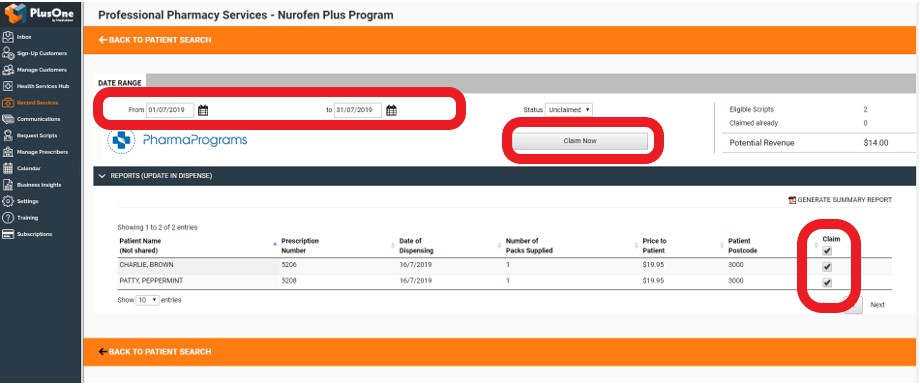This image is a screenshot from a website called "Plus One," which offers professional pharmacy services, specifically the Neurofen Plus Program. The interface has a blue sidebar on the left side, featuring various tabs, although the text is too small to read clearly. At the top of the main section, there is an orange bar with an arrow labeled "Back to Patient Search."

Beneath this bar, there is a "Date Range" section showing a range of dates from January 2019, though the exact dates are not clear. Following that, there are headings "Pharma Programs" and "Status: Unclaimed," accompanied by a "Claim Now" button highlighted in red. The section also indicates "Eligible Scripts: 2," "Claimed Already: 0," and "Potential Revenue: $14,000."

Below this summary, there is a detailed table listing the patients. The table includes columns for patient name, prescription number, date of dispensing, number of packs supplied, price to patient, and patient postcode. Notably, there is a section circled in red labeled "Claim," with three checkboxes, all of which are checked.